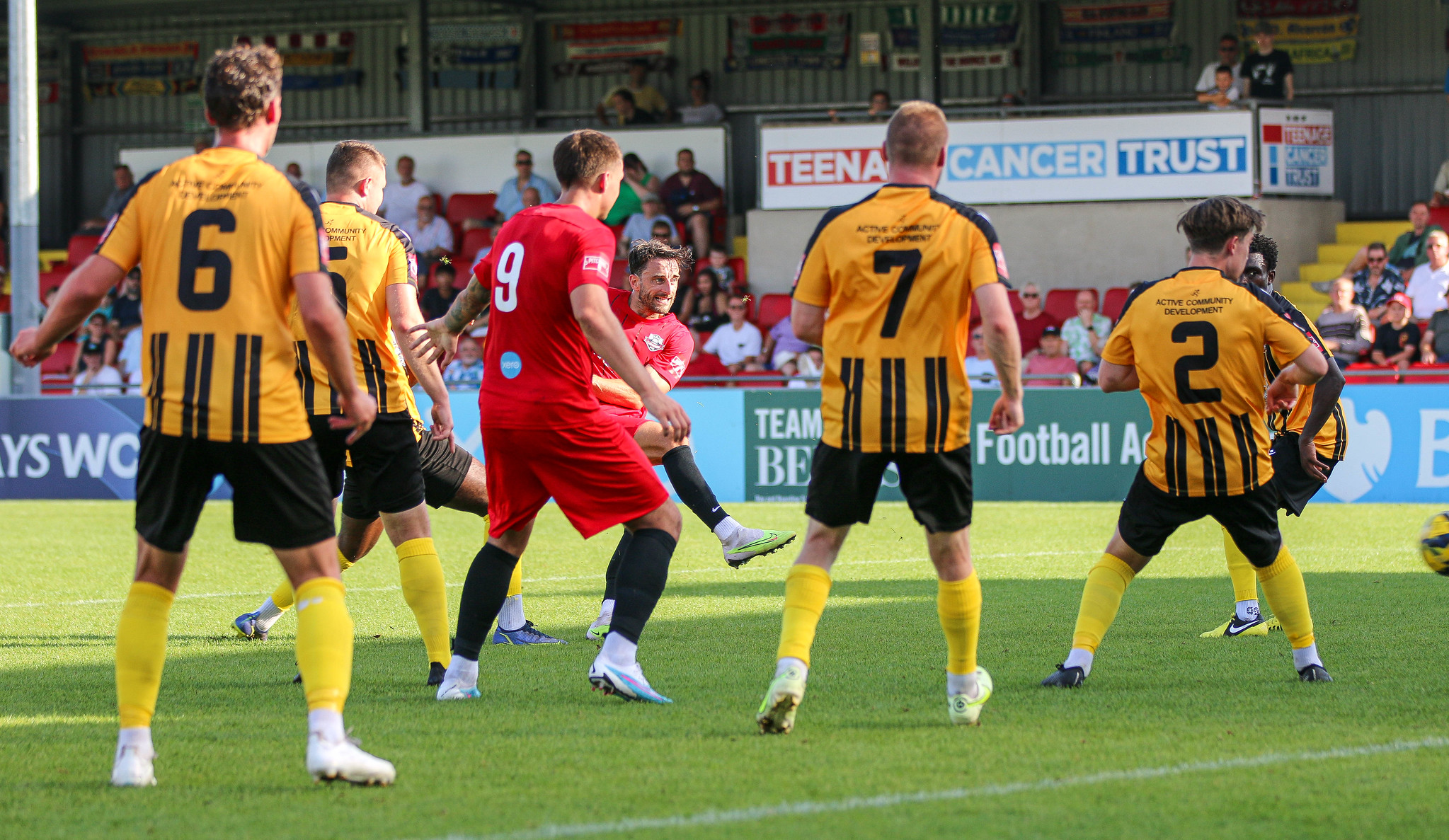The photograph captures an outdoor soccer match between two teams. The team in yellow shirts with black stripes and black shorts features players with numbers 6, 5, 7, and 2 visible. The opposing team is clad in red shirts and shorts, with number 9 noticeable, and another player just having kicked the ball, which is yellow and blue. In the background, a crowded spectator stand is filled with fans, and the seats are colored yellow and red. Surrounding the field are various advertisements, including a partially visible sign promoting the Teenage Cancer Trust and another ad beginning with "Bar." A blue fence borders the field, adding to the vibrant ambiance of the scene.